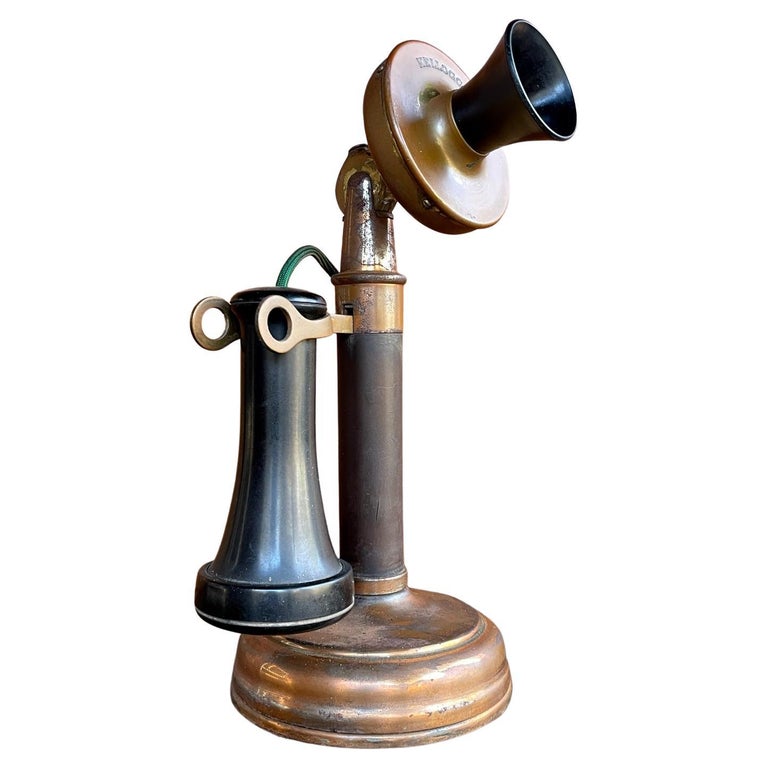This image showcases an artist's detailed rendition of a historic, early model telephone set against a white background. The antique phone, most likely from the late 1800s or early 1900s, features a unique two-part design distinct from modern-day receivers. The mouthpiece, a gold speaker with a black opening, is affixed atop a cylindrical rod that extends down to a gold-plated base. The listening piece, resembling a bell shape or a salt shaker, hangs upside down, captured between two ornate gold prongs attached to the side. This ear piece, with its broader black base tapering toward the top, rests on a holder linked to the mouthpiece by a cord. Notably, there are no dial numbers present on this pedestal-type phone, emphasizing its early technological design. This beautifully crafted collectible would attract antique enthusiasts and serves as a nostalgic reminder of the early days of telecommunication.